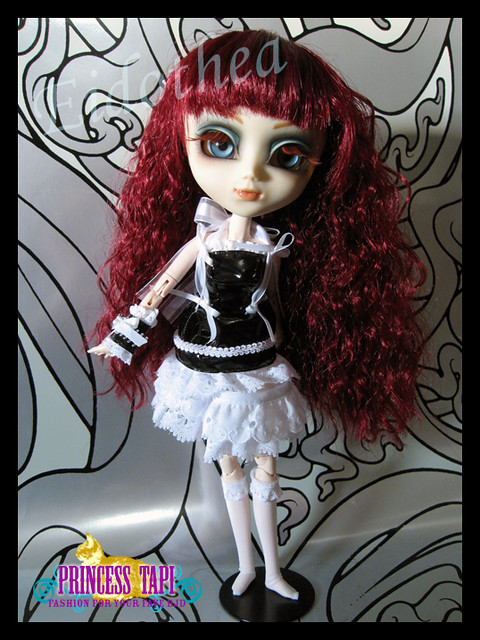In this detailed photograph, a doll resembling a Bratz character is prominently featured against an abstract, silver and black backdrop with curvy patterns and a combination of light gray areas. The doll sports long, curly red hair that extends all the way down to her legs, complemented by straight bangs. Her distinct features include pale skin, extraordinarily large blue eyes with red eyelashes, and orange eyebrows. She has a notably slender neck and arms, making her head appear disproportionately large. Her attire consists of a black and white ruffle dress adorned with ribbons and see-through sleeves, similar to a French maid's costume. She pairs this with knee-high, sheer white socks with lace and ruffles. The doll stands on a black, round platform supported by a little stand. In the lower left-hand corner of the image, text reads "Princess Toppy" atop a gold cat, followed by an illegible line that suggests a fashion theme.